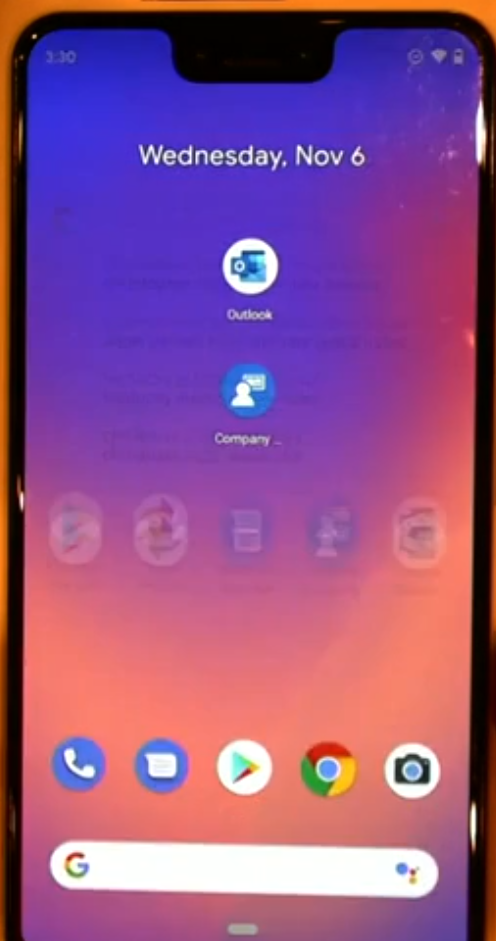The image depicts the front view of a cell phone with its screen lit up, captured by an external camera. The image is blurry, resulting in some elements appearing overlapped and doubled. The display shows the date as Wednesday, November 6th. Below the date, there are two partially discernible icons - one for Outlook and the other presumably for a company. Further down, five indistinct icons are visible, but due to the blurriness, their functions are unclear. Clearer towards the bottom, there are five specific icons: a call button, a messaging button, the Google Play Store logo, the Google Chrome logo, and a camera icon. At the very bottom, there is a search bar with the Google logo. The phone's background features an abstract blend of blue, purple, pink, and orange shades, layered in various patterns across the screen.